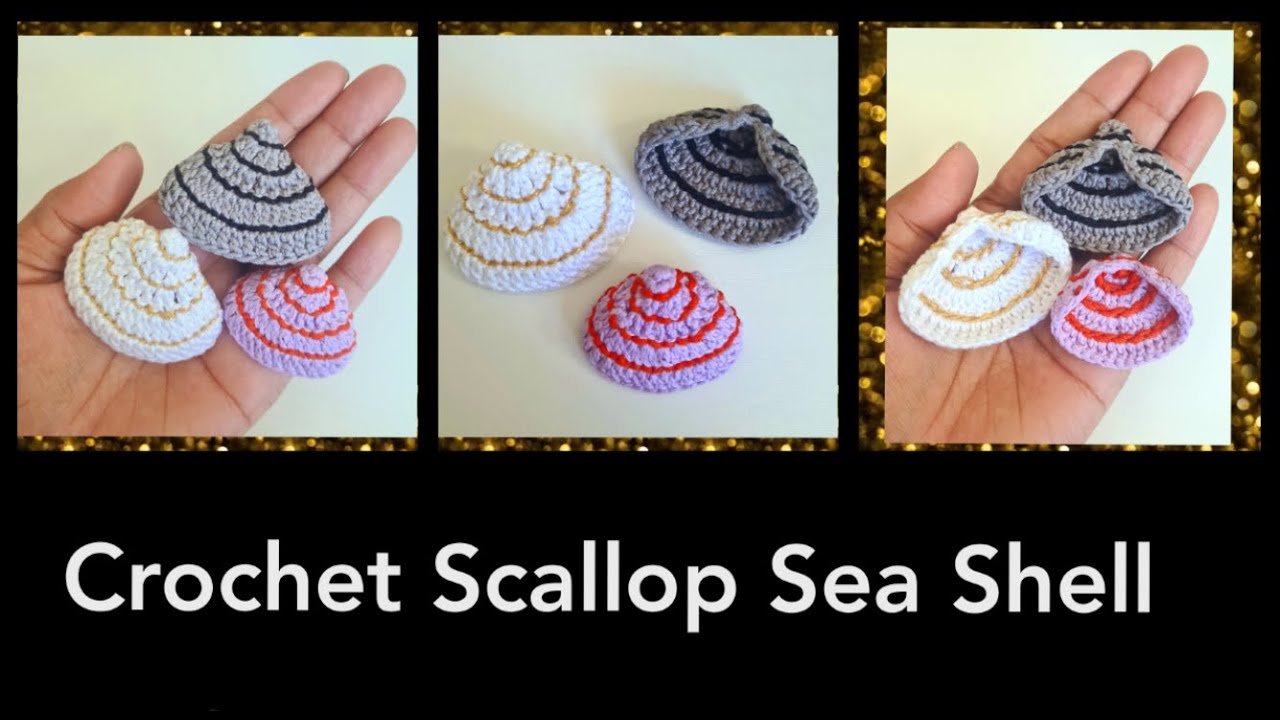The image features a striking triptych of crocheted scallop seashells, arranged in a horizontal line against a sleek black background. The outer frames are adorned with glittering gold borders, adding an extra touch of elegance. At the bottom of the series, the words "crochet scalloped seashell" are displayed in clean white text. 

In the first and third pictures, a hand is seen holding the seashells. In the first image, the hand holds them right side up, while in the third image, they are presented upside down, showcasing their intricate details. The middle image focuses solely on the seashells without the hand, offering a clear view of their craftsmanship.

The seashells themselves come in three distinct color patterns: one is grey with black concentric rings, another is white adorned with orange rings, and the third is a delicate light purple with striking red lines. The careful arrangement and detailed representation highlight the beauty and artistry of the crocheted seashells, making this a visually captivating piece.